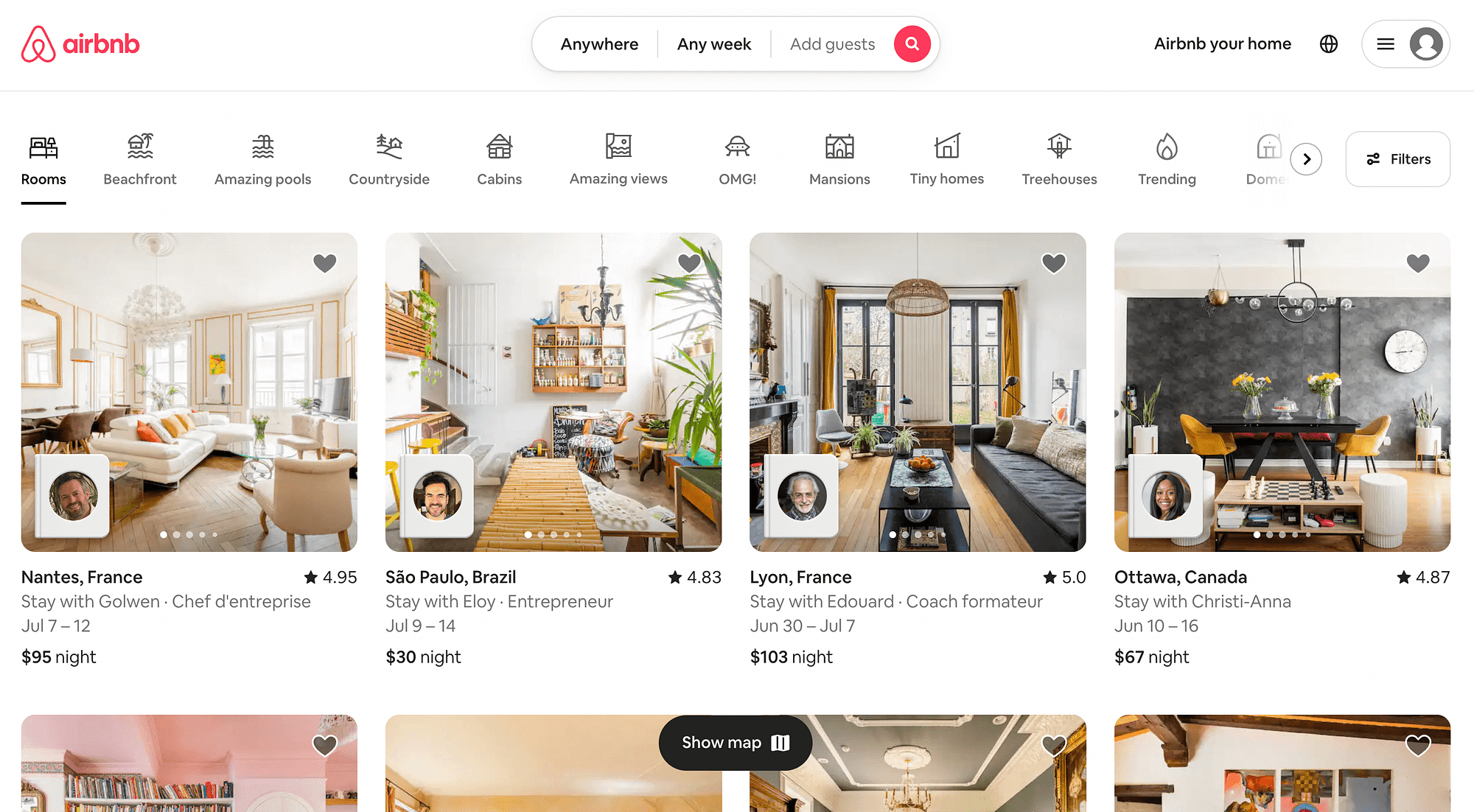The image depicts a screenshot of the Airbnb website interface. 

### Detailed Caption:

The Airbnb website is prominently displayed, beginning with the iconic red Airbnb logo situated at the top left of the screen. Centered at the top is a navigation bar featuring three circular nodules. Each nodule is labeled with black, bold text: "Anywhere" on the left, "Any Week" in the middle, and a grayed-out "Add Guests" on the right, accompanied by a red magnifying glass icon. 

Directly below, a horizontal strip showcases approximately eleven icons, suggesting quick access or filtering options. At the end of this strip, a "Filters" bar is visible, setting the stage for the detailed listings below.

The foremost row of listings presents various rental options, each complete with an eye-catching image. The properties include:
1. A room in Nantes, France priced at $95 per night.
2. A room in Sao Paolo, Brazil available for $30 per night.
3. A luxury option in Lyon, France costing $103 per night.
4. A comfortable rental in Ottawa, Canada for $67 per night.

Each listing includes a thumbnail image of a person on a small notebook icon, presumably representing the host or the type of accommodation. Below these primary options, the edge of the image shows four additional listings, each partially visible.

At the bottom of the screen, a "Show Map" button appears in a black bar with white text and an integrated icon, inviting users to explore the available accommodations on a map for better geographic context.